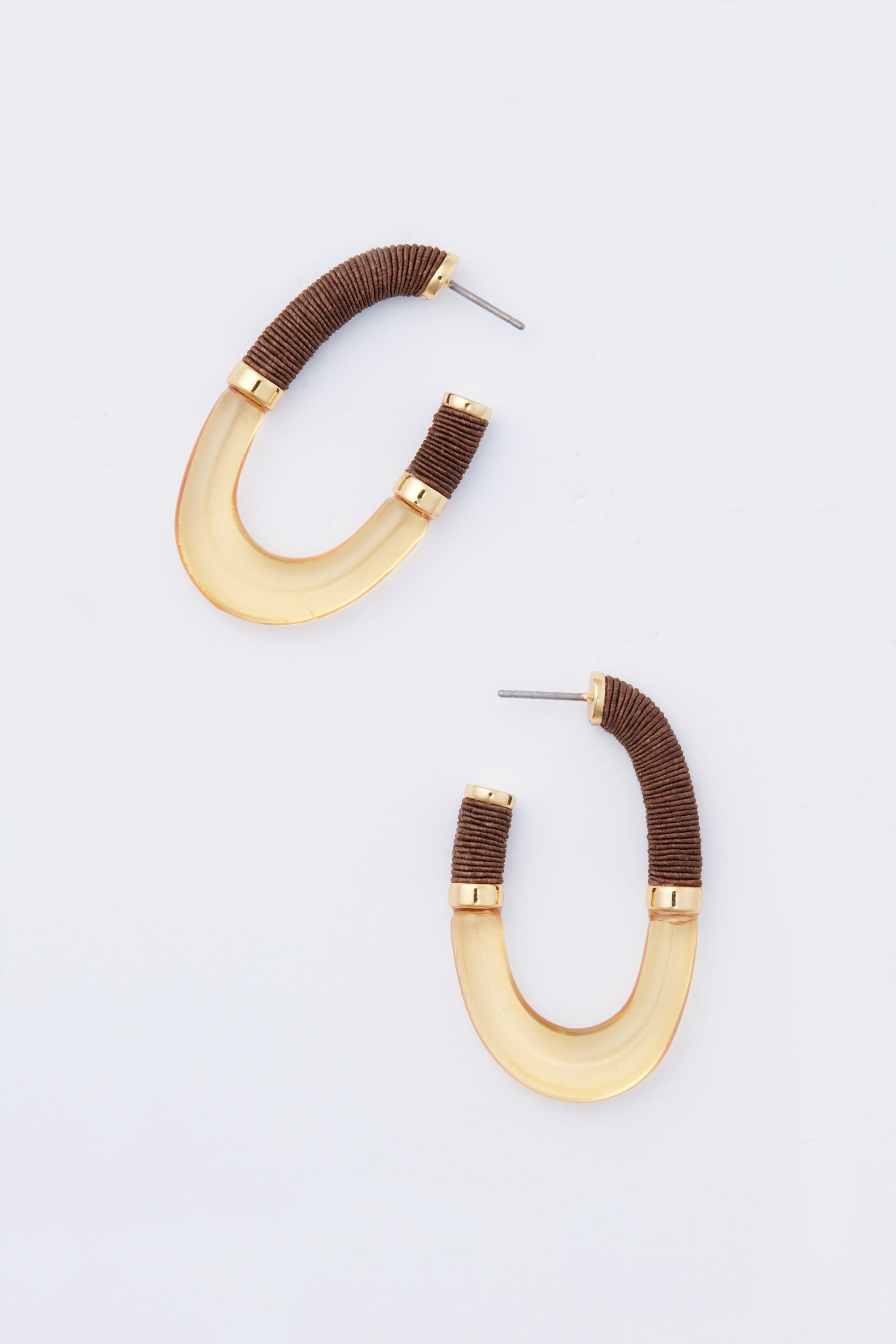This close-up image captures a single pair of earrings, likely ear studs intended for pierced ears, showcased against a light gray background. The earrings feature a protruding metal pin, indicative of their design meant to go through the earlobe. Each earring has a half-spherical shape with an intricate design. The upper section of the earring is a light yellow-brown, resembling half a moon or sphere, and appears to have an irregular texture, possibly resembling wrapped thread or an artsy style design. This section is contrasted with gold bands that separate it from the bottom portion of the earring, which is a clear, whitish beige. The combination of the brown and whitish beige sections, along with the golden bands, gives the earrings an elegant and stylish look.